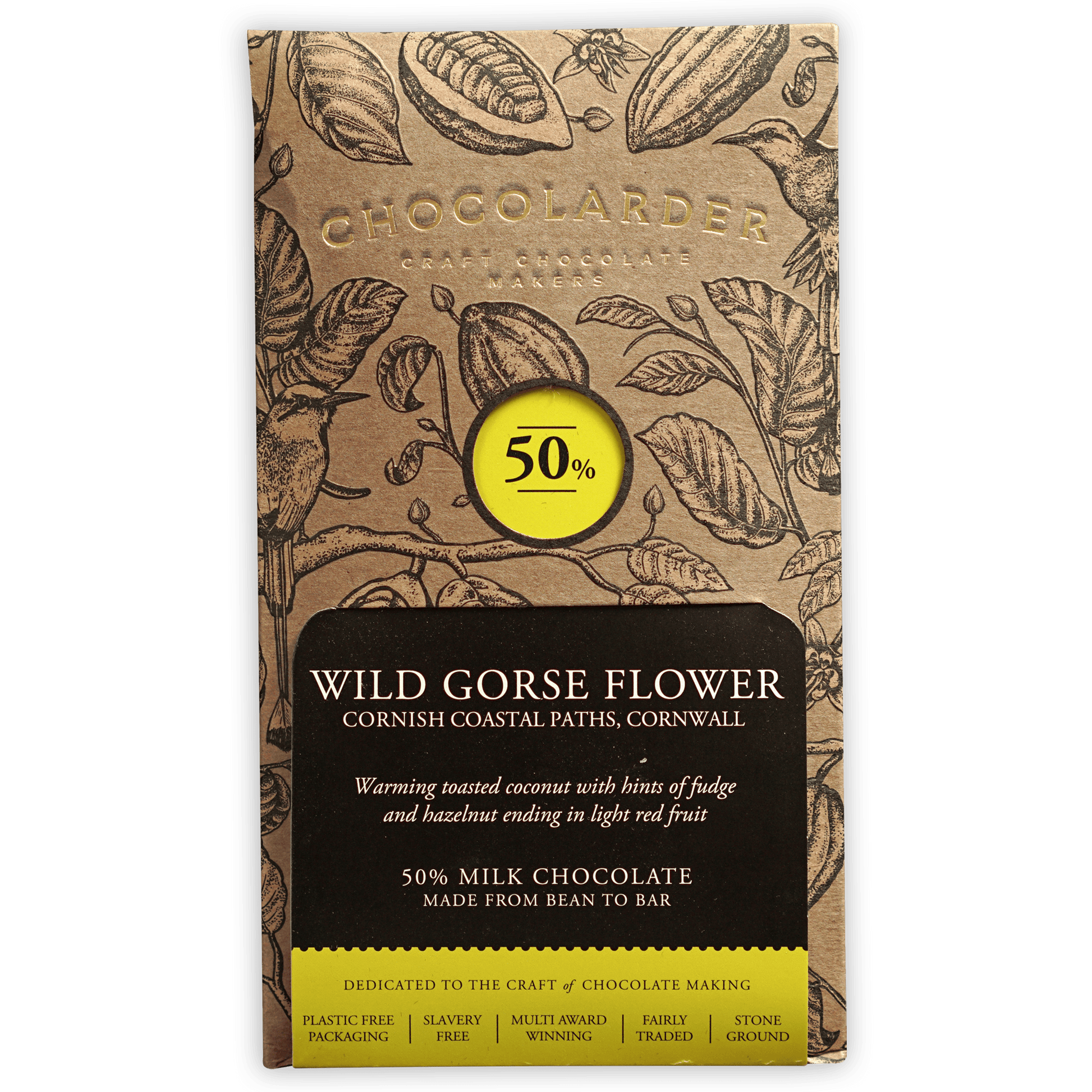The image showcases a sophisticated chocolate product encased in a gold copper-colored paper packaging. The product is a vertically shaped, beige chocolate bar. At the top of the packaging, the brand name "Chocolarder" is prominently displayed in a slightly hard-to-read beige text against the background, followed by "Craft Chocolate Makers." Below this, a distinct yellow circle highlights the text "50%" which indicates the chocolate is made up of 50% milk chocolate. The intricate design on the packaging features delicate illustrations of branches and leaves, along with a tastefully included bird motif. The label also states "Wild Gorse Flower, Cornish Coastal Pass, Cornwall," suggesting both the origin and the unique ingredients of the chocolate. The bar promises a sensory experience with "warming toasted coconut with hints of fudge and hazelnut ending in light red fruits." This carefully crafted chocolate bar, made from bean to bar, underscores the artisanal quality and minimal processing involved in its creation.